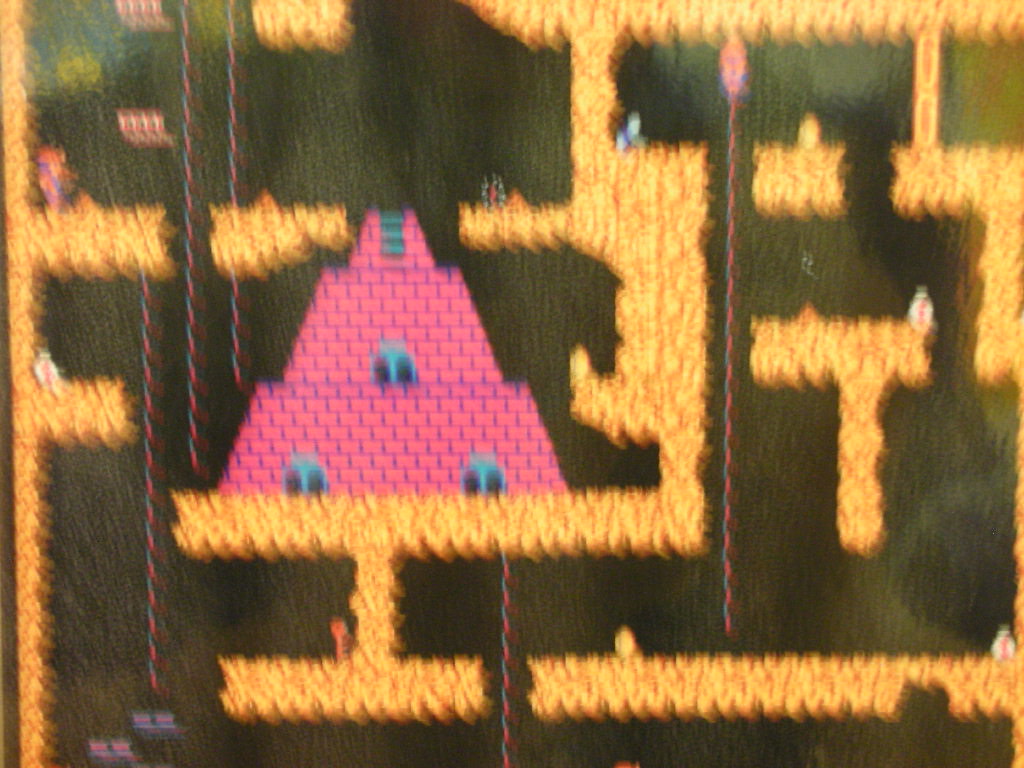This image appears to be a blurry photograph of a vintage arcade video game, likely from the early to mid-1980s. The primary focus is a large, pink pyramid-like structure with horizontal layers, which is positioned on yellowish-golden sand-like elements. The pyramid features two blue windows at the bottom, one middle window, and a small ladder or rack near the top. The background is black, enhancing the vivid colors of the game elements. Various pink, white, and peach icons are scattered across the screen, including snowman-shaped icons and streamer-like ropes in pink and blue on either edge. On both sides of the image, tiny person-like icons can be seen, one on each side, including a figure in the upper left possibly wearing a miner’s helmet, though the image is blurry. The layout suggests a vertical pathway filled with obstacles, reminiscent of a game like Donkey Kong.